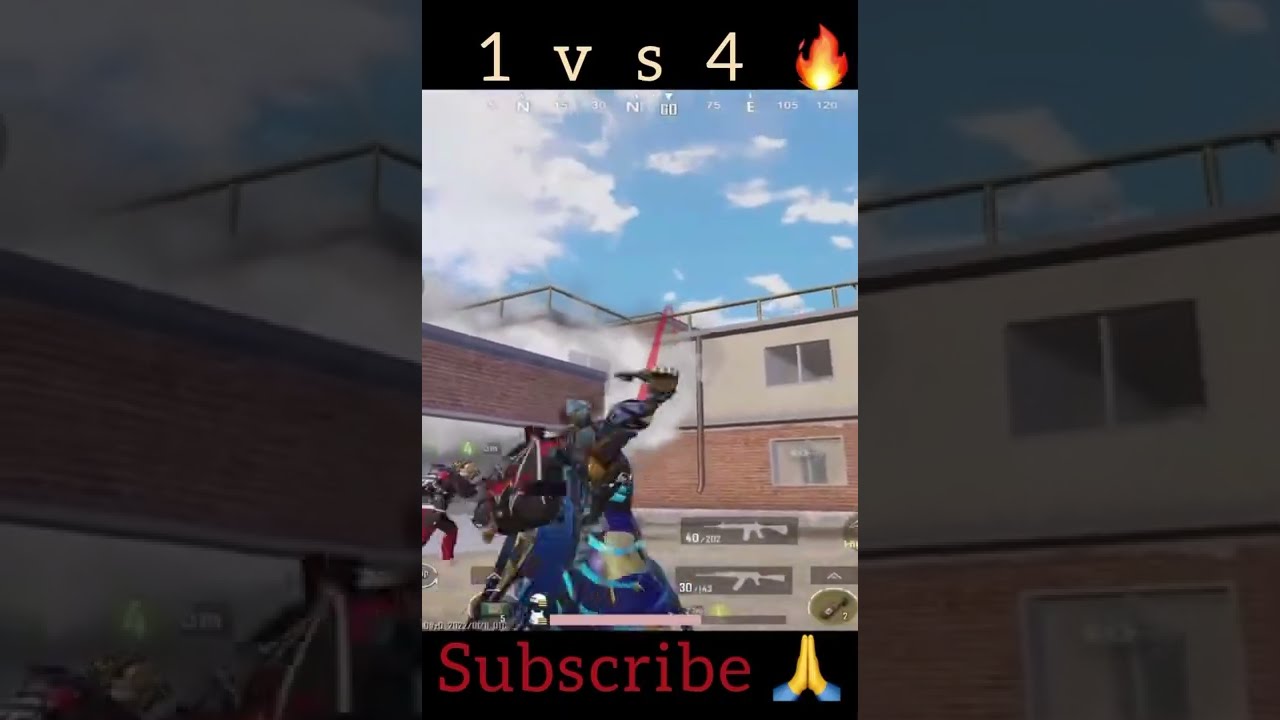The image is a highly detailed, stylized screenshot that resembles a scene from a video game or comic book. It's a vertical, rectangular photo framed by faded, zoomed-in versions of the same scene on its left and right edges. At the top of the central image, there's a black bar occupying the top eighth of the photo, containing the text "1v4" followed by a red flame emoji. Directly below, a crisp blue sky with puffy white clouds sets the scene over a two-story commercial building, white on the top floor and orangey on the bottom, with windows dotting its facade. 

In the lower left of the frame, there appears to be a combat situation, though the details are somewhat blurred. Two characters, one in blue and black robes and possibly mounted on a horse, are engaged in what looks like a fight. Further in the background, more characters can be discerned, adding to the chaos of the scene.

At the bottom, another black bar stretches across, displaying the text "subscribe" in red letters. Accompanying this text is an emoji of two pale hands pressed together in a prayer gesture. Additionally, the presence of a compass direction with 'N' and 'E' along with an indicator of weapons and remaining ammunition adds to the sense that the viewer is witnessing a moment from an action-packed video game.